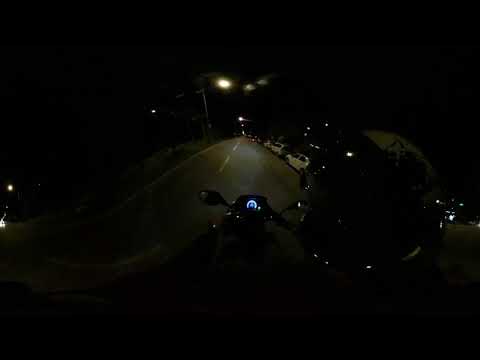In this night-time photograph, taken from the first-person perspective of someone riding a motorcycle, the scene is enveloped in darkness. The dimly lit instrument panel is visible, heightening the sense of nocturnal adventure. The headlight of the motorcycle provides the primary source of illumination, casting a beam along a two-lane roadway that extends into a vanishing point on the horizon. The middle of the road is marked with visible stripes, guiding the rider forward. A few light-colored cars are parked on the right side of the road, adding hints of life to this solitary journey. Scattered throughout the image are small lights, likely from distant street lamps and other vehicles, speckling the darkness. On the left-hand side, an additional light glows faintly against the inky sky. The image captures the essence of a lone ride through the night, with the road and its subtle details coming alive through the focused beam of the motorcycle's headlight.